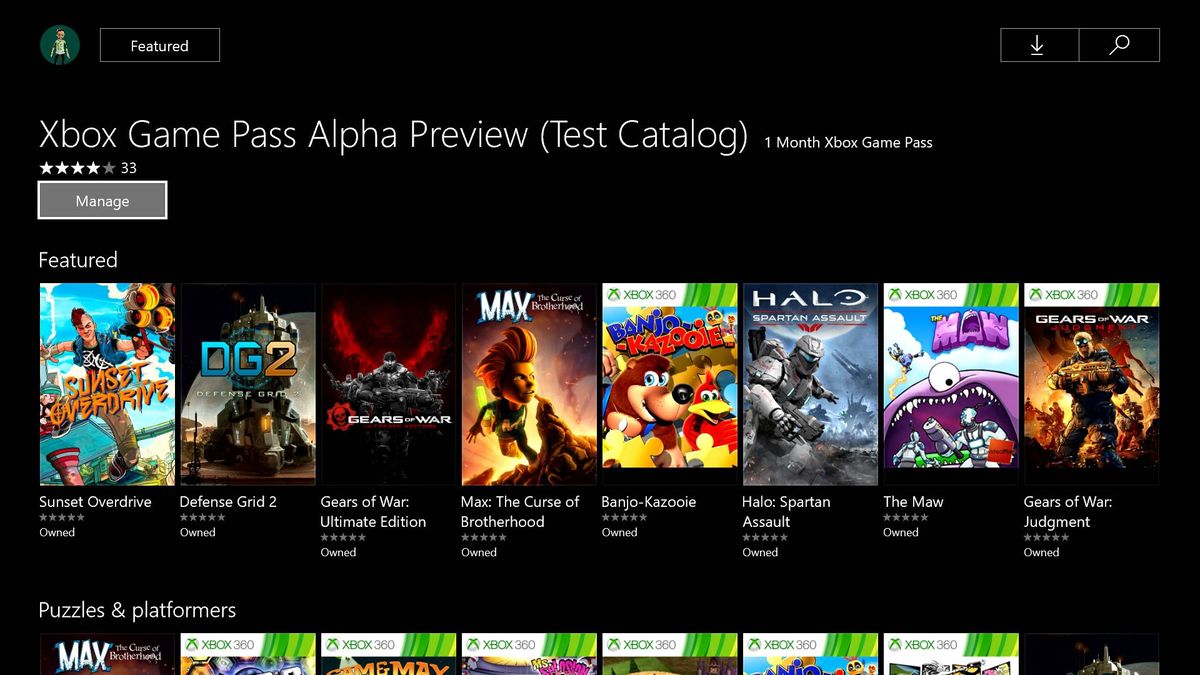This image showcases the Xbox Game Pass Alpha Preview Test Catalog interface. In the top left corner, there is an account icon. Adjacent to it in the top right corner are a square download icon and a square search magnifying glass icon. The title, "Xbox Game Pass Alpha Preview Test Catalog," is prominently displayed along with the subscription duration, "One Month Xbox Game Pass."

Beneath the title, there is a "Manage" button, and a gray box containing a 4-star rating. Below, a featured games section displays a list of titles:

1. Sunset Overdrive
2. Defense Grid 2
3. Gears of War: Ultimate Edition
4. Max: The Curse of Brotherhood
5. Banjo-Kazooie
6. Halo: Spartan Assault
7. The Maw
8. Gears of War: Judgment

Additionally, the bottom row of the game list includes "Puzzle Pirates," but it is slightly cut off, making other titles partially visible yet unreadable. The overall background of the interface is black. Under the Xbox Game Pass Alpha Preview Test Catalog heading, a star rating of 4 out of 5, based on 33 ratings, is displayed.